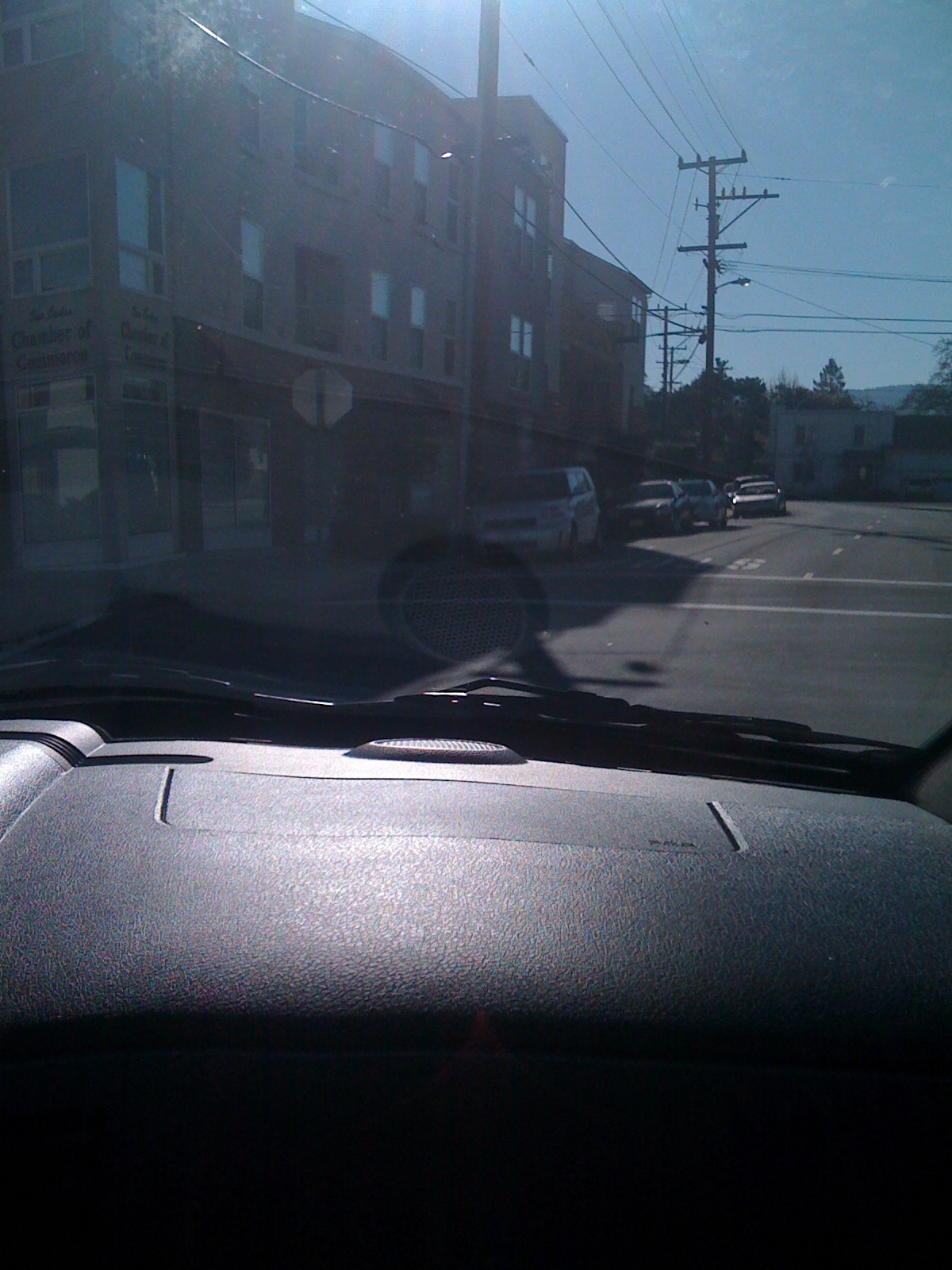The image captures a scene from the passenger side of a vehicle with a dark interior, likely black, filling up about 40% of the frame. The photo is oriented in a vertical manner, which emphasizes more height than width. Through the windshield, the top of the right windshield wiper is visible, along with some glare on the window, indicating the sun is high in the sky, casting beams of light. The road ahead appears straight but veers slightly to the right, suggesting the car might be positioned slightly to the left of the street's centerline.

On the left side of the road, there is a distinctive three-story brick corner building with the words "Chamber of Commerce" in block letters, though the top words are unreadable. Other buildings of varying heights are also present. Several vehicles, approximately four to six, are parked on the left side of the road, facing the opposite direction, hinting at a possible one-way street or opposite-facing parking regulations. Telephone poles and wires run alongside the buildings, and a house can be seen in the distant background. Furthermore, there is a reflection on the dashboard, suggesting the presence of the sun. The dashboard also includes elements like an airbag indentation and a speaker below the windshield.